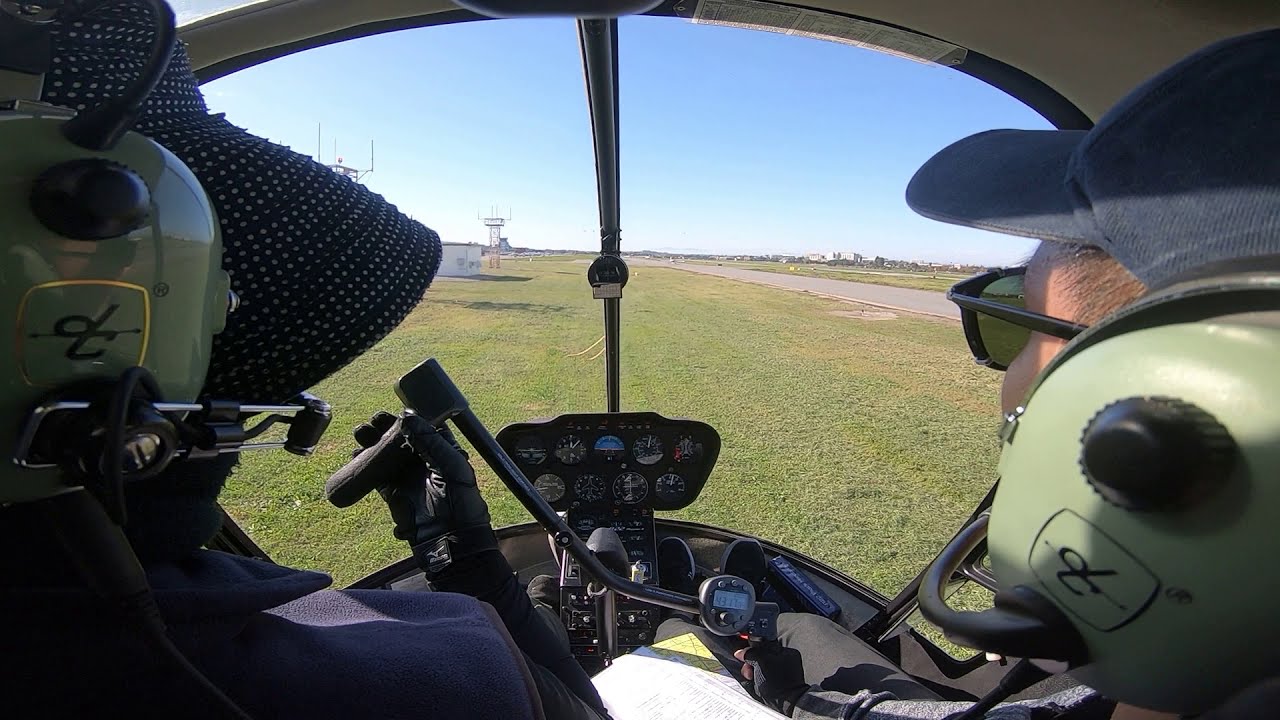The photograph, taken from the rear interior of a helicopter cockpit on a sunny day, captures two individuals seated in the front seats, both facing an open green field with a long paved runway to the right. The person on the left, wearing a black bonnet with white polka dots, black gloves, and beige-colored headphones, sits alongside the person on the right, who is equipped with a blue baseball cap, sunglasses, and identical headphones. They both tend to a black control panel brimming with various circular gauges and dials, some of which likely include a timer, evidencing their aviation expertise. The clear blue sky above the horizon adds to the scene's serene yet professional ambiance.